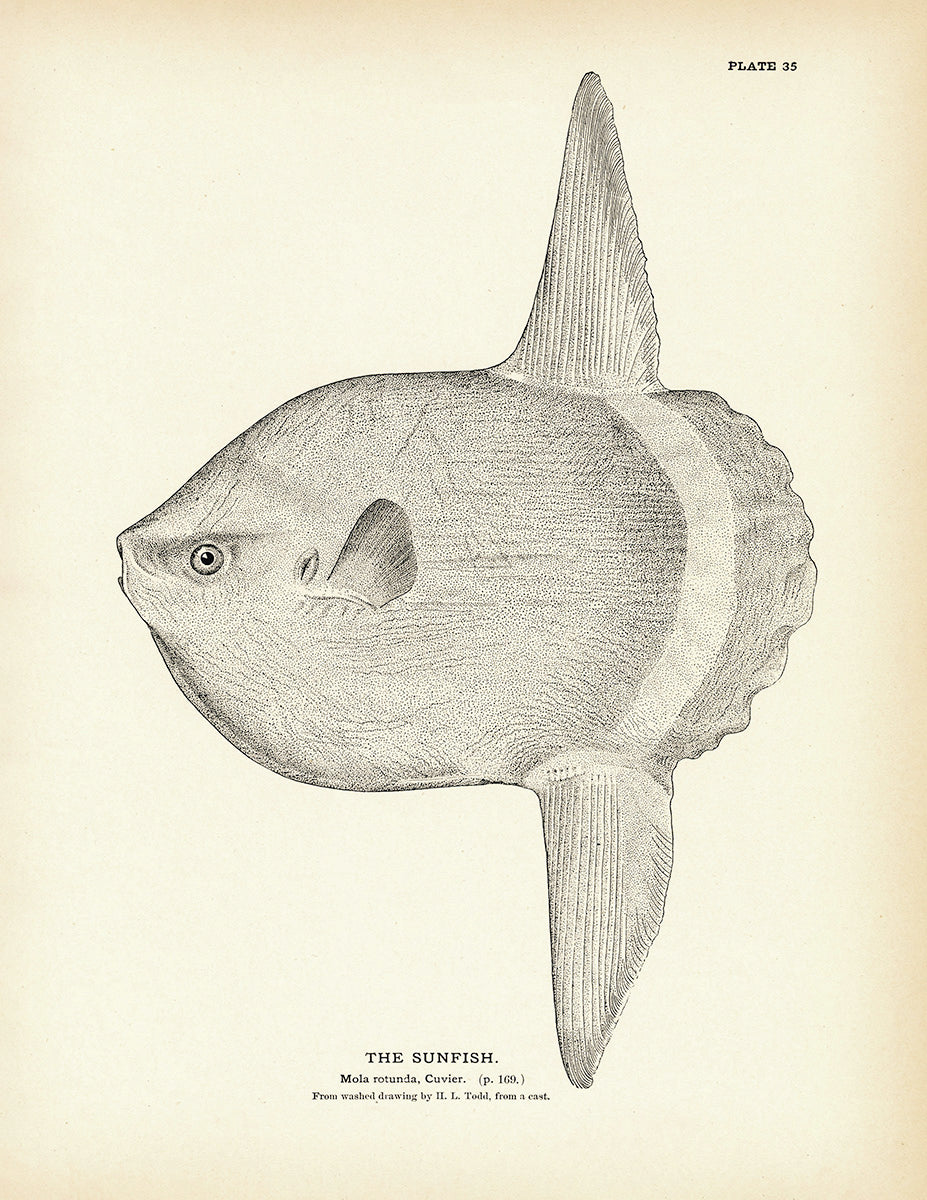This detailed black and white pencil drawing of a sunfish is set against a light beige or light pink background. The composition is vertical, about one and a half times as tall as it is wide. The prominent text in the upper right corner reads "Plate 35." 

The drawing captures the unique shape of the sunfish, characterized by its large, oval body. It features a pointy nose at the left end, a small, puckered mouth, and a round, bright eye just behind a small fin. The sunfish's distinctive fins extend both upward and downward from the center of its body—both fins are triangular with visible vertical lines. A subtle yet noticeable white stripe curves across the fish’s body, connecting the top and bottom fins.

Additional text at the bottom of the image reads, "The Sunfish. Mola, Rotunda, Cuvier," followed by "P.169" in parentheses, and a note beneath that which appears to say, "From Washed Drawing by H.T. Todd," though this part is difficult to read. The finely detailed pencil work highlights the fish's bumpy, curved back and small gills, capturing the essence of its aquatic form.